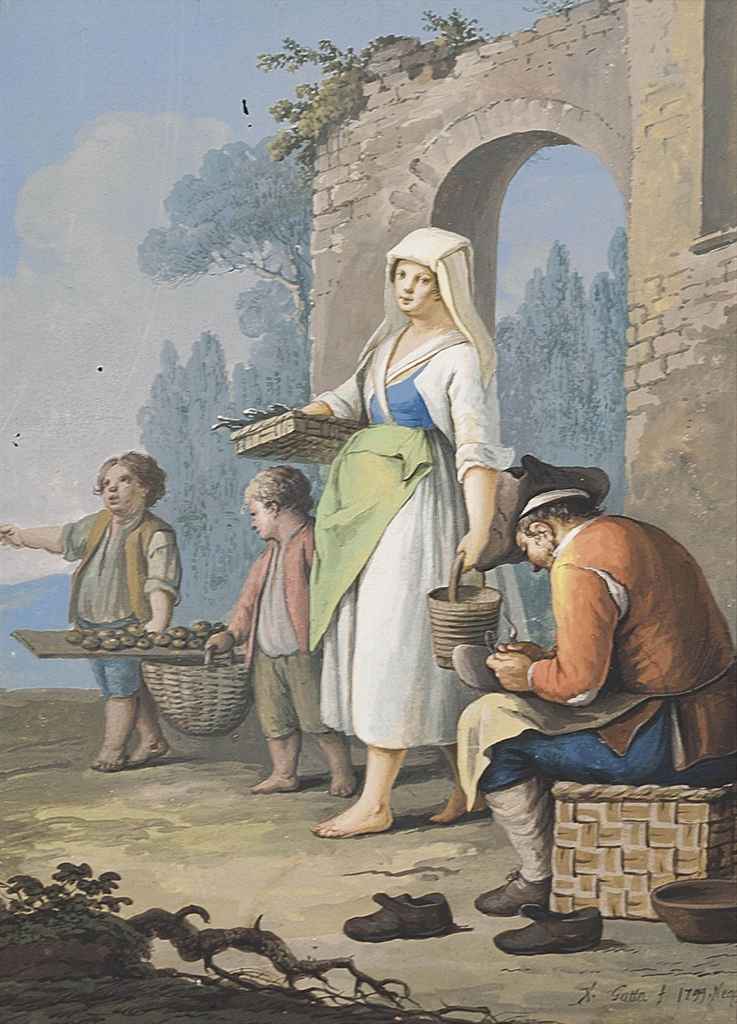This detailed Renaissance-style painting captures a colorful and vibrant medieval scene set against a backdrop of a European brick villa with an archway, possibly in Italy or France. The central figure is a woman in her 30s, wearing a white dress with hints of blue underneath a green apron, complemented by a white scarf around her head. She gracefully balances a bucket in her left hand and a flat basket possibly filled with vegetables or fish in her right arm. 

Accompanying her are two barefoot children dressed in gray shirts and vests—one in a pink vest and blue shorts, the other in a beige vest and beige shorts—who share the task of carrying a basket and a board adorned with what seems to be potatoes or similar produce. They appear to be heading towards a market.

On the side, a seated man, possibly the father, is depicted as a cobbler mending a shoe. He dons a dark tricorn hat, a beige jacket with visible wear and tear, a beige apron, blue pants, white socks, and gray shoes. The scene includes additional shoes scattered on the floor, suggesting his craft.

The atmosphere is pastoral and serene, characterized by soft pastel colors, towering trees in the background, and a clear blue sky dotted with white clouds.